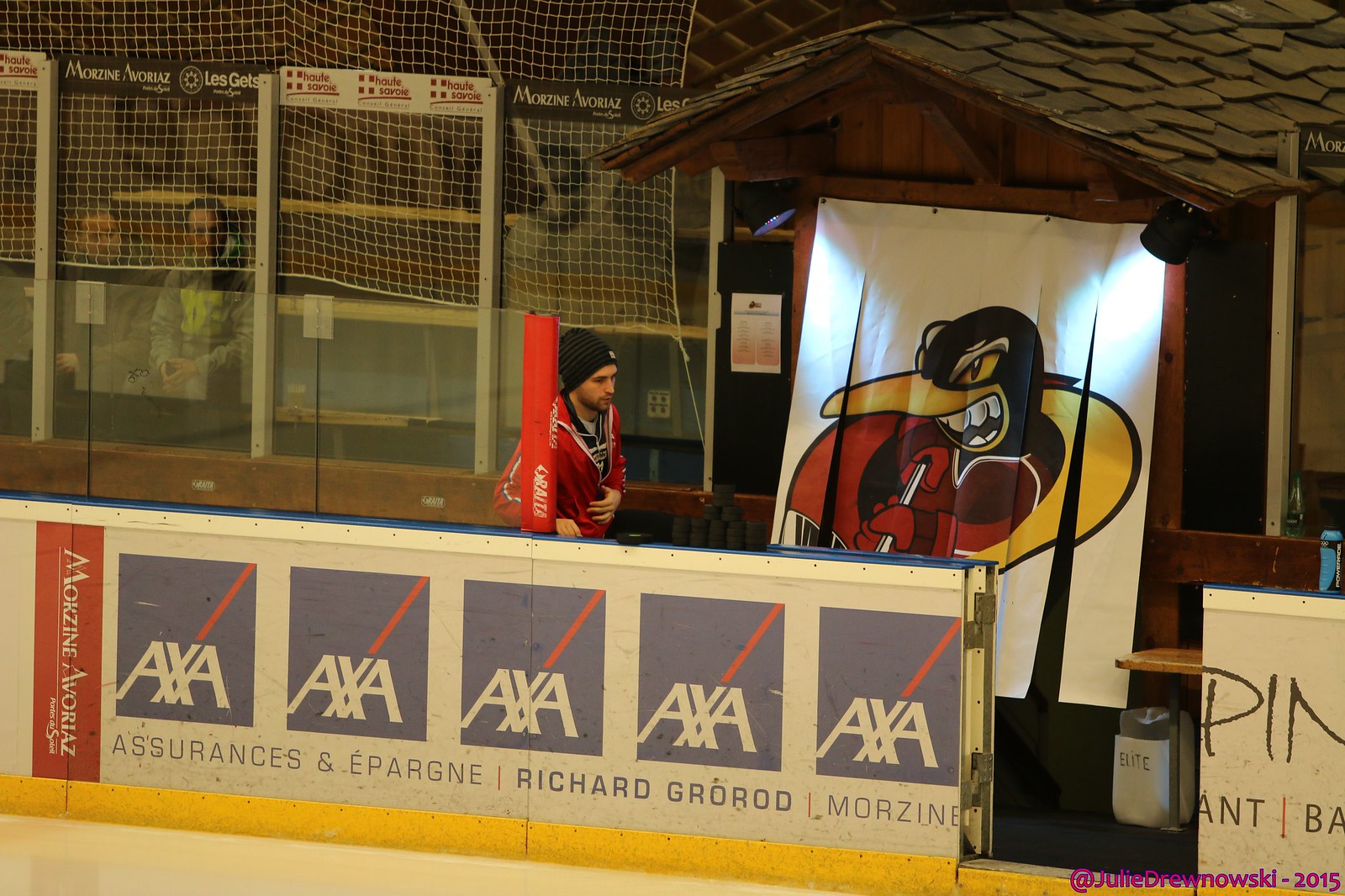This photograph captures a detailed scene inside a bustling hockey arena. Dominating the image is a hockey player, seen from the waist up, approaching a set of open doors that lead onto the rink. The player is decked out in a distinctive red jersey and wears a black beanie. To the right of the player, the door is open, revealing a glimpse of the ice rink in the lower left-hand corner. The walls surrounding the player are a combination of white, yellow at the base, and topped with blue trim. Adorning these walls are various blue and red logos and advertisements, including one that reads "Moczine Evoriates," among other phrases, such as "Assurances" and "Iparn Richard Grorard Moczine." A striking banner above the player depicts an angry black bird with a yellow beak and a red jacket. The bird imagery sits atop a small structure resembling a hut with shingles. On the upper left-hand corner, netting covers some glass walls, beyond which blurred figures of fans are visible, adding to the lively atmosphere of the arena. At the bottom right-hand corner of the image, a section of the advertisement reads, "At Julie Drew Nowski 2015," grounding the photo in a specific time and place.